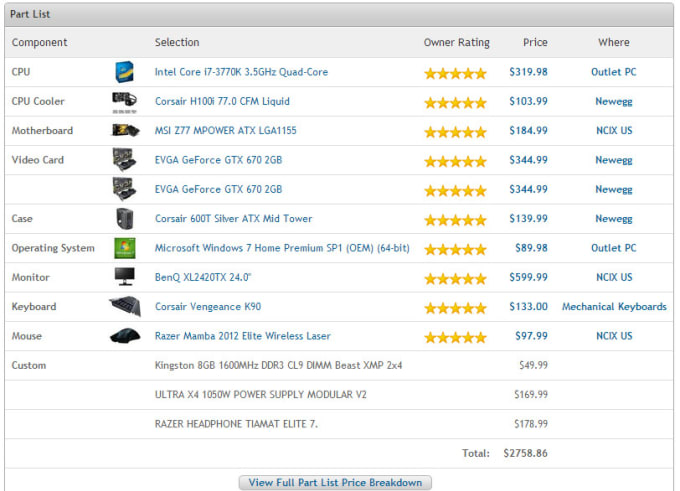This image appears to be a computer screenshot featuring a "Part List," most likely sourced from an online retailer or a PC building website. It showcases a table against a white background with a slightly gray border outlining the entire image. At the top of the image, a gray bar spans the width, indicating the title "Part List" situated in the upper left corner.

Below the gray bar, the table is organized into multiple columns with the following headings: "Component," "Selection," "Owner Rating," "Price," and "Where." 

- The first entry under "Component" is labeled "CPU," accompanied by a thumbnail image of a blue and yellow box, indicating an Intel product. The "Selection" field details it as an "Intel Core i7 Quad-Core Processor," highly rated with "5 stars." The price is listed at "$319.98," and the item is available from "Outlet PC."
  
- Another entry for the "Case" component features a representation of a black box, specified as a "Corsair 600T Silver ATX Mid Tower." This product also receives a "5 stars" rating, is priced at "$139.99," and is available from "Newegg."

Overall, this part list is a breakdown of various computer components complete with their specific details, owner ratings, prices, and the stores where they can be purchased. The information is presented in a structured format, making it clear and easy to comprehend for someone looking to build or upgrade a PC.